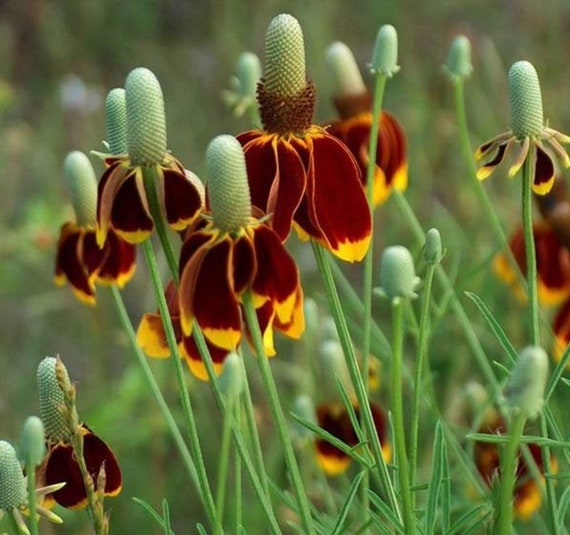The image captures a close-up view of several flowers in a natural setting. The flowers, which number around ten, exhibit drooping maroon and crimson petals, often tipped with yellow or purple. The petals point downward towards the center, where there are large green buds that resemble small cacti with a bumpy texture and sometimes brown fuzz near their bases. The foreground is densely populated with these flowers and their stems, some of which lack petals and feature small, green, pill-shaped buds. Surrounding the flowers are long, crisscrossing blades of grass. The background remains out of focus, hinting at more flowers and grass, contributing to a slightly gloomy yet serene daytime scene in the wild.